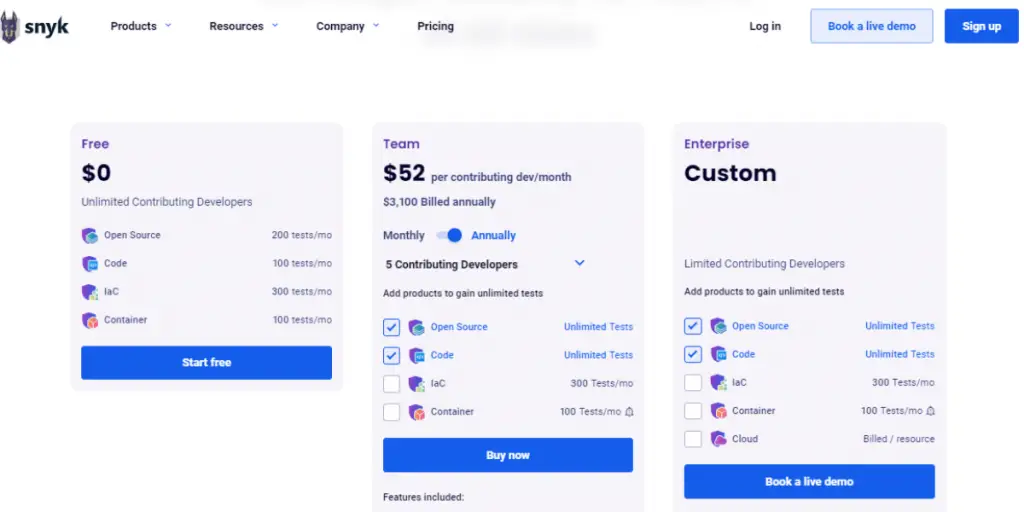This is a detailed caption for the described image from the SNYK website:

---

The image is a long rectangular screenshot of the SNYK website. In the top-left corner, there's the SNYK logo, which features a stylized dog emblem in a grayish-purple hue, accompanied by "SNYK" written in black letters.

To the right of the logo is a navigation bar featuring several sections, each followed by a downward-pointing gray "V" symbol indicating drop-down menus: "Products," "Resources," "Company," and "Pricing." On the far right of the navigation bar, the black letters "Login" are visible, followed by a blue rectangle with white letters inside that read "Book a live demo." To the right of this button, there are the words "Sign up" in blue letters, and a blue box with white letters inscribed "Sign up."

Below the navigation bar, three pricing option boxes are displayed horizontally:

1. **First Box (Smallest)**:
   - **Header**: In purple letters, it shows "$0".
   - **Text**: Below, it states "unlimited contributing developers" in gray letters, followed by numerous statistics related to open source code, IAC, container, and other icons which are not clearly identifiable.
   - **Stats**: It mentions "200 tests/MO" and similar metrics.
   - **Button**: At the bottom, there is a large blue bar with "Start Free" written in white letters.

2. **Middle Box (Medium Size)**:
   - **Header**: The word "Team" in purple, followed by "$52" per contributing developer per month in black letters.
   - **Pricing Details**: Indicates "$3,100" billed annually, with an option to toggle between monthly and annually, currently set to annually.
   - **Features**:
      - "5 contributing developers"
      - "Add products to gain unlimited tests"
   - **Options**:
      - "Open Source" and "Code" are checked with blue checkmarks, offering unlimited tests.
      - "IAC" and "Container" are unchecked with options like "300 tests/MO" and "100 tests/MO" underneath.
   - **Button**: A blue box with "Buy Now" in white letters, and below it, "Features included" in black, although part of this text is cut off.

3. **Third Box (Largest)**:
   - **Header**: "Enterprise" in purple letters.
   - **Text**: Below, "Custom" in black letters with a significant gap between them and additional content.
   - **Details**:
      - Mentions "limited contributing developers"
      - "Add products to gain unlimited tests"
   - **Options**:
      - "Open Source" and "Code" are checked with blue checkmarks, indicating unlimited tests.
      - "IAC," "Container," and "Cloud" are unchecked with various indeterminate statistics.
   - **Button**: A large blue box with "Book a live demo" in white letters.

---

This caption provides a comprehensive overview of the screenshot from the SNYK website, detailing each element and section within the image.